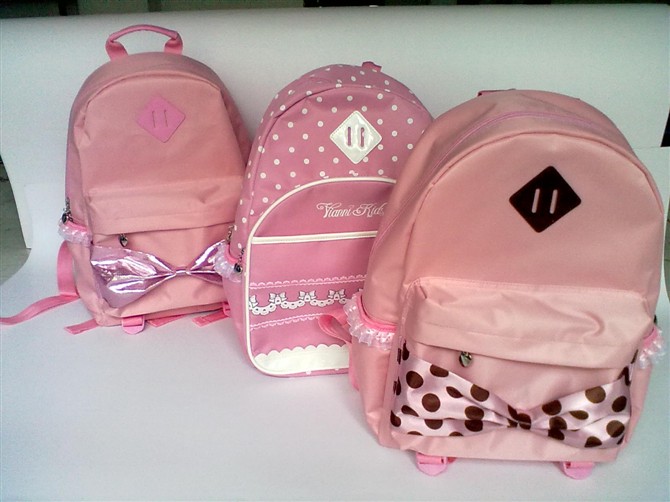The photograph depicts three pink backpacks positioned vertically on a white chair, against a white background. The chair itself features a seat and a straight backrest. The backpacks are slightly overlapping each other. 

On the left, the first backpack is light pink with a shiny, metallic pink bow attached to the front zipper pouch, which is highly reflective and likely crinkly in texture. The handle of this backpack is also pink.

The middle backpack is a darker shade of pink, adorned with white polka dots on the upper portion. It features a front zipper pouch with an intricate lacy design and a silver diamond detail at the top.

The backpack on the right is a solid pink with a silky, light pink bow covered in brown polka dots at the bottom. It also has a lace-like fabric around the circumference of its front zipper pouch.